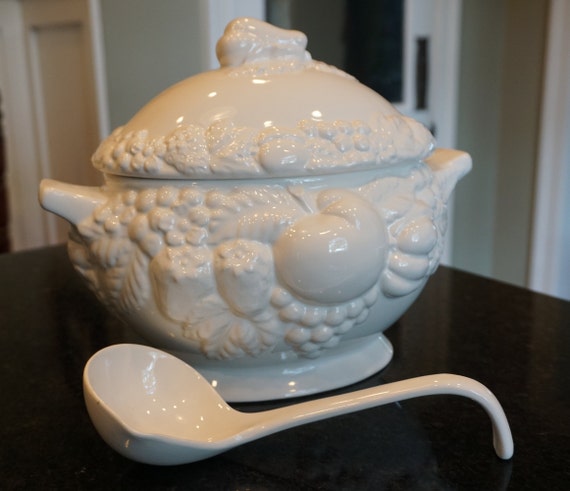This photo features a large, vintage white glazed ceramic soup tureen, elegantly resting on a dark wooden table. The oval-shaped tureen, complete with a matching lid and a substantial base, boasts an intricate relief design of various fruits—grapes, apples, strawberries, and grape leaves—encircling both the bowl and the lid. The tureen is equipped with two handles on either side for easy transport. Accompanying the tureen is a coordinating white ladle, characterized by a large scoop and a gracefully curved handle, positioned prominently in the foreground. The background reveals a homely setting with neutral tones, enhancing the timeless charm and excellent condition of this mid-century serving piece.